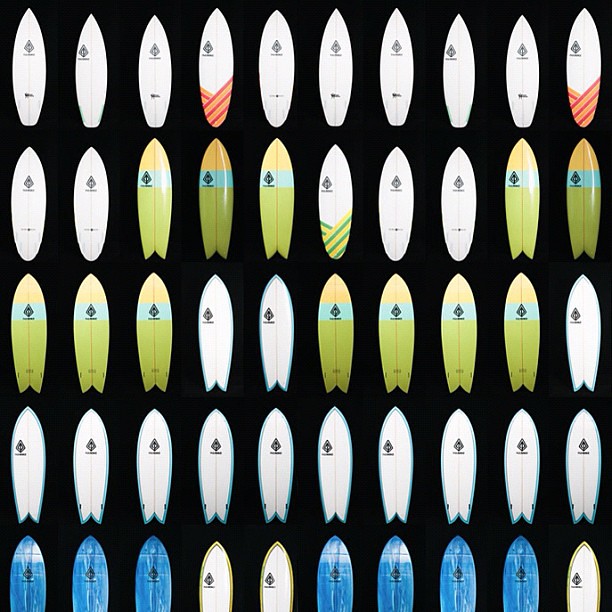This image displays a meticulously arranged grid of surfboards against a black background. There are five rows with ten surfboards each, viewed from a top-down perspective. The surfboards, predominantly white, feature a distinctive black logo resembling a diamond with a shorter bottom section. A pattern emerges throughout the collection: the first row includes mostly white boards with two exhibiting a light and dark orange striped design. The second row shows a blend, primarily of white surfboards and several green ones transitioning to yellow at the tip. The middle row consists of three white surfboards followed by seven having the same green-to-yellow gradient. The fourth row returns to an assortment of primarily white surfboards with the black emblem prominently displayed. At the bottom, the surfboards are largely blue with a few white ones interspersed. This cohesive but colorful array suggests a uniform branding, possibly from the same company, represented by the consistent logo on each board.